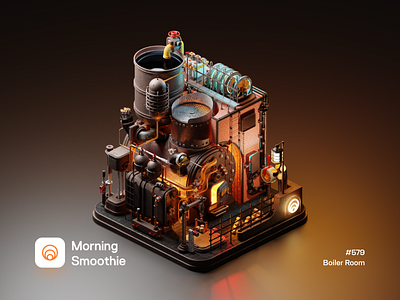The image is a detailed depiction of what appears to be a 3D-rendered boiler room or a highly detailed scale model of one, identified as "Morning Smoothie, number 579, boiler room." The centerpiece of the image is a complex and meticulously crafted boiler unit featuring various mechanical components: a main boiler with an open furnace door illuminating a dark red glow, multiple vats including one with a dark liquid and another with a lid, and an assortment of interconnected pipes. Blue discs, surrounded by metal rings, sit atop the structure, which is encased in wood metal panels edged with metal borders. 

The setup features walkways, control levers (one with a red winch), and a grey fuse box emitting a blue glow. A single lantern, made of black metal, adds subtle lighting to the scene. The structure is seen against a plain gradient background shifting from brown to gray, enhancing the focus on the central mechanical composition. The image also includes a logo with concentric circles on the bottom left, labeled "Morning Smoothie," and the text "579 boiler room" on the right, reinforcing the fictional and stylized nature of the depiction.